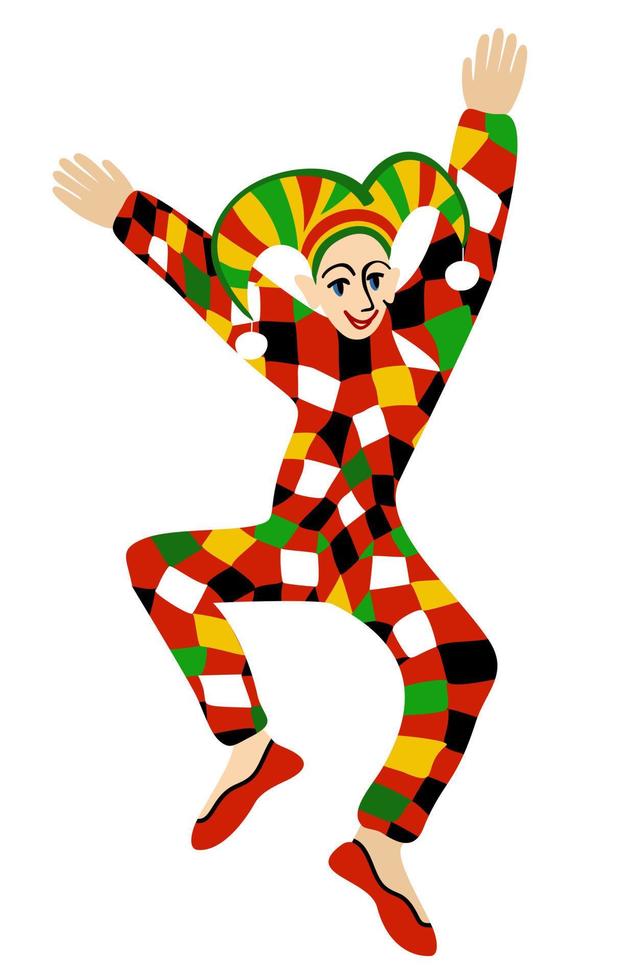This image is a graphic illustration, reminiscent of a children's book, depicting a cartoonish, flat, two-dimensional jester in mid-dance. The jester's hat has two fronds in alternating stripes of yellow, green, and red, tipped with white pom-poms. They sport a colorful jumpsuit adorned with a patchwork of squares in red, white, black, green, and gold. The jester's expressive face features blue eyes and pointy red lips forming a wide smile. Their arms are exuberantly raised above their head, while their legs are spread apart as if jumping joyfully. The jester completes the lively scene with bright red shoes.